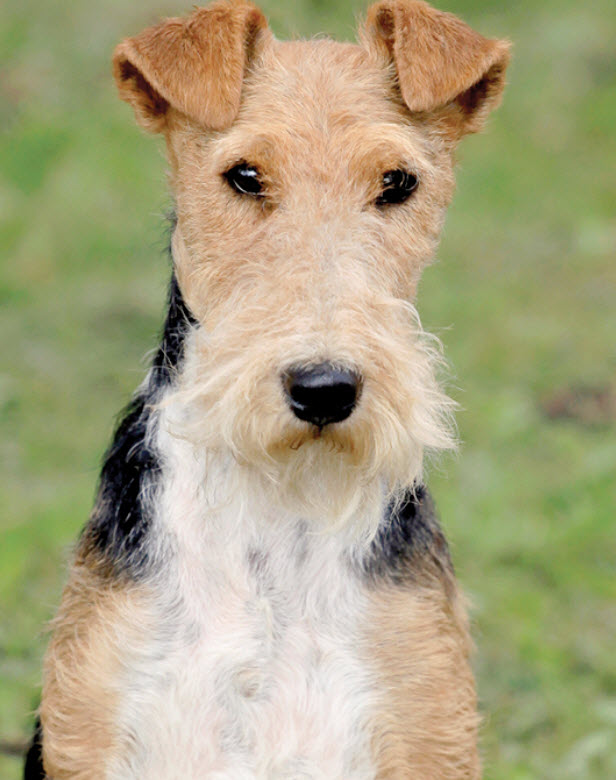This image features a dog sitting calmly and staring directly into the camera, with a backdrop of green, grassy turf. The dog has a distinctive, wire-haired coat and displays a mix of brown, black, and white fur. His face is light brown, with darker brown, woolly-textured ears that are folded over at the top. His eyes and nose are strikingly black. Around his mouth, white fur extends below his lips, giving the impression of a mustache. A black fur pattern resembling a cape covers the back of his neck and stops at his shoulders, blending with his white chest. His legs, beneath his shoulders, are a light khaki tan. The dog's composed expression and medium-length fur contribute to his content appearance.